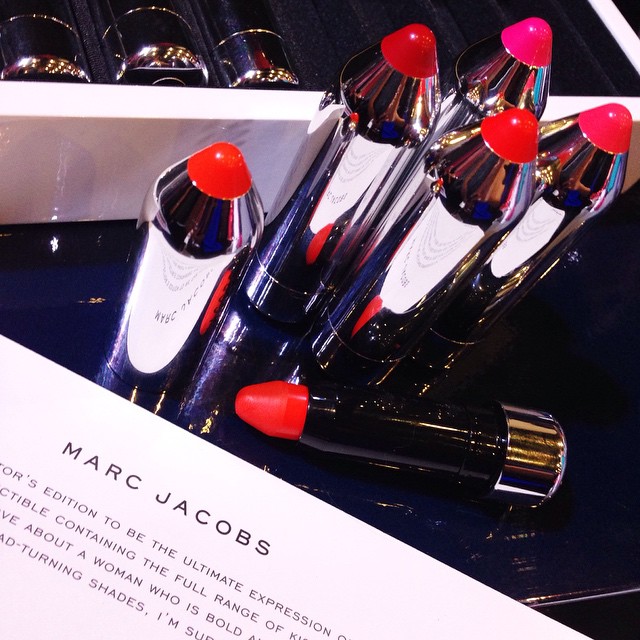The image showcases a tilted photograph of six shiny silver lipstick dispensers arranged on a blue surface. Five of the lipsticks stand upright, their bright red tips visible, while a sixth lies on its side in the foreground. The interior of the tubes is black, contrasting with the vibrant lipstick color. A partially visible white card with black text in the bottom left corner spans diagonally across the image, reading "Marc Jacobs" and fragments of phrases like "addition to be the ultimate expression," "containing the full range," "about a woman who is bold," and "head-turning shades." Above the lipsticks is a case displaying three more lipstick containers, with additional slots on the right, emphasizing the elegance and comprehensive nature of the collection.